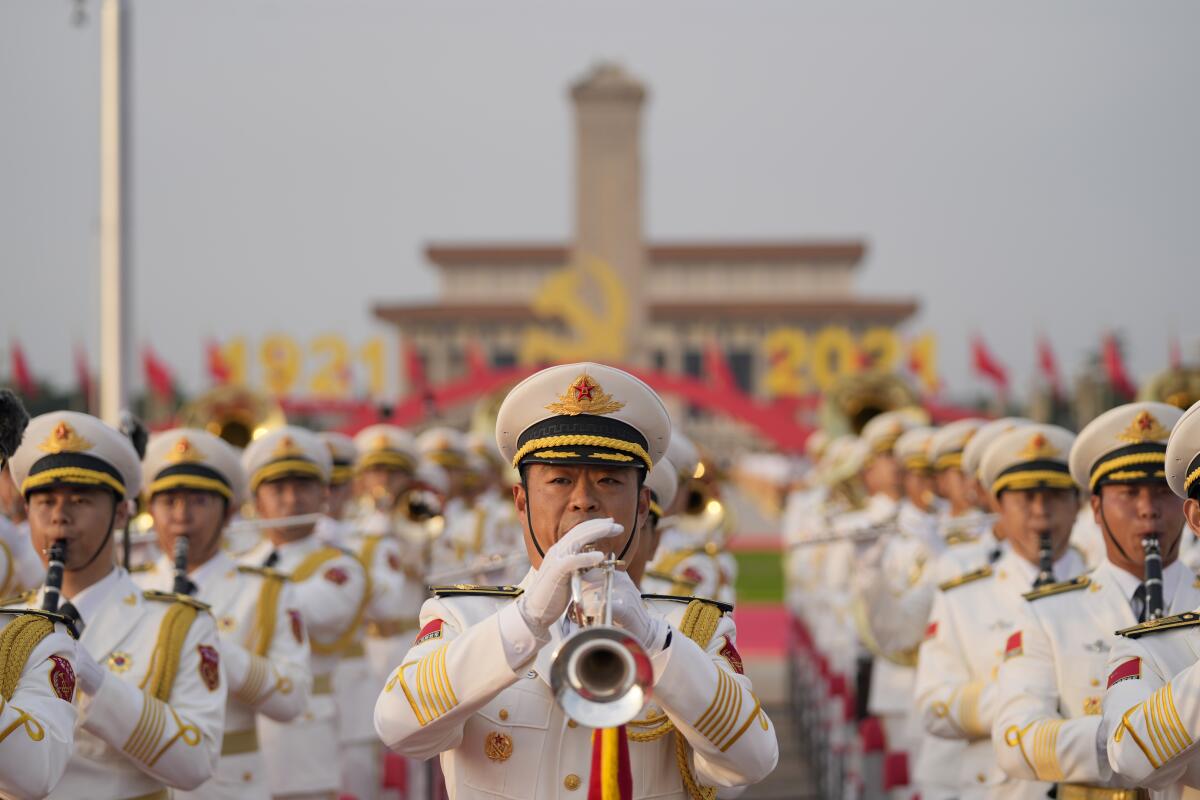The photo captures an outdoor scene of an organized parade, likely at a festival or ceremonial event, featuring a group of musicians dressed in military-style uniforms. The men, who appear to be Asian, are all aligned in tight formation, each wearing predominantly white uniforms accentuated with gold and red highlights. Their hats, also white, bear a striking gold emblem with a red star. The focus of the image is on a central figure playing a trumpet, flanked by others with various wind instruments. All musicians sport white gloves, with their jackets displaying ornate gold and red accents, including distinctive bands across the lower sleeves. The background reveals a complex setting with numerous red flags, a 2021 numerical display, and a prominent gold hammer and sickle, suggesting a communist theme, possibly indicative of the Soviet Union or similar state. Additionally, there is a tall brown building with a tower, blurred but visible, under a clear blue sky with green and red elements on the ground.